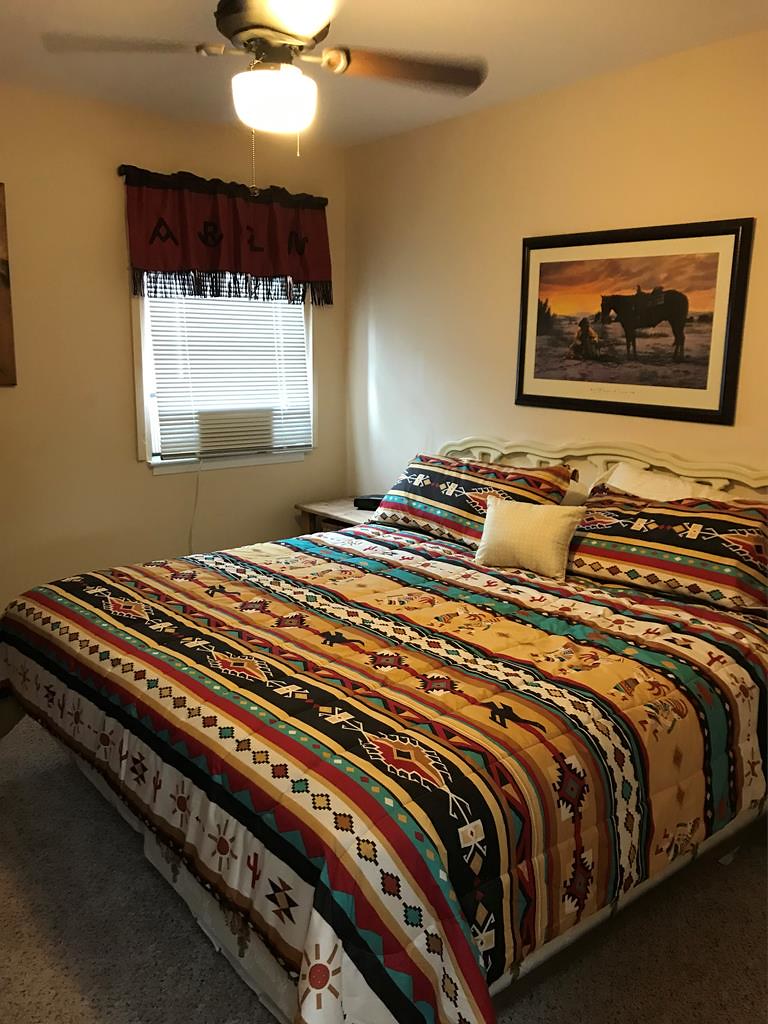The photograph captures a tidy and inviting bedroom. Dominating the room is a large bed, possibly queen-sized, covered with a vibrant bedspread featuring an intricate Southwestern or Native American-inspired pattern. The multicolored bedspread showcases an array of geometric designs and motifs, including cacti, suns, and tribal elements, primarily in shades of red, yellow, black, and teal. At the head of the bed, matching pillows flank a smaller, plain white cushion, and plain white pillows provide additional contrast.

The room is illuminated by a ceiling light with a fan, casting a warm, cozy glow. A window in the upper left corner has white Venetian blinds fully drawn and is topped with a reddish-brown valance with decorative black accents. The walls are a neutral beige color, contributing to the room's serene atmosphere, and the floor is carpeted in a matching beige tone.

Above the bed hangs a prominent framed painting featuring a horse by a kneeling or squatting Native American figure set against a sunset backdrop. The black frame of the painting ties the visual elements together, adding to the room's cohesive aesthetic. Overall, the scene portrays a well-organized and aesthetically pleasing bedroom with a strong Southwestern theme.